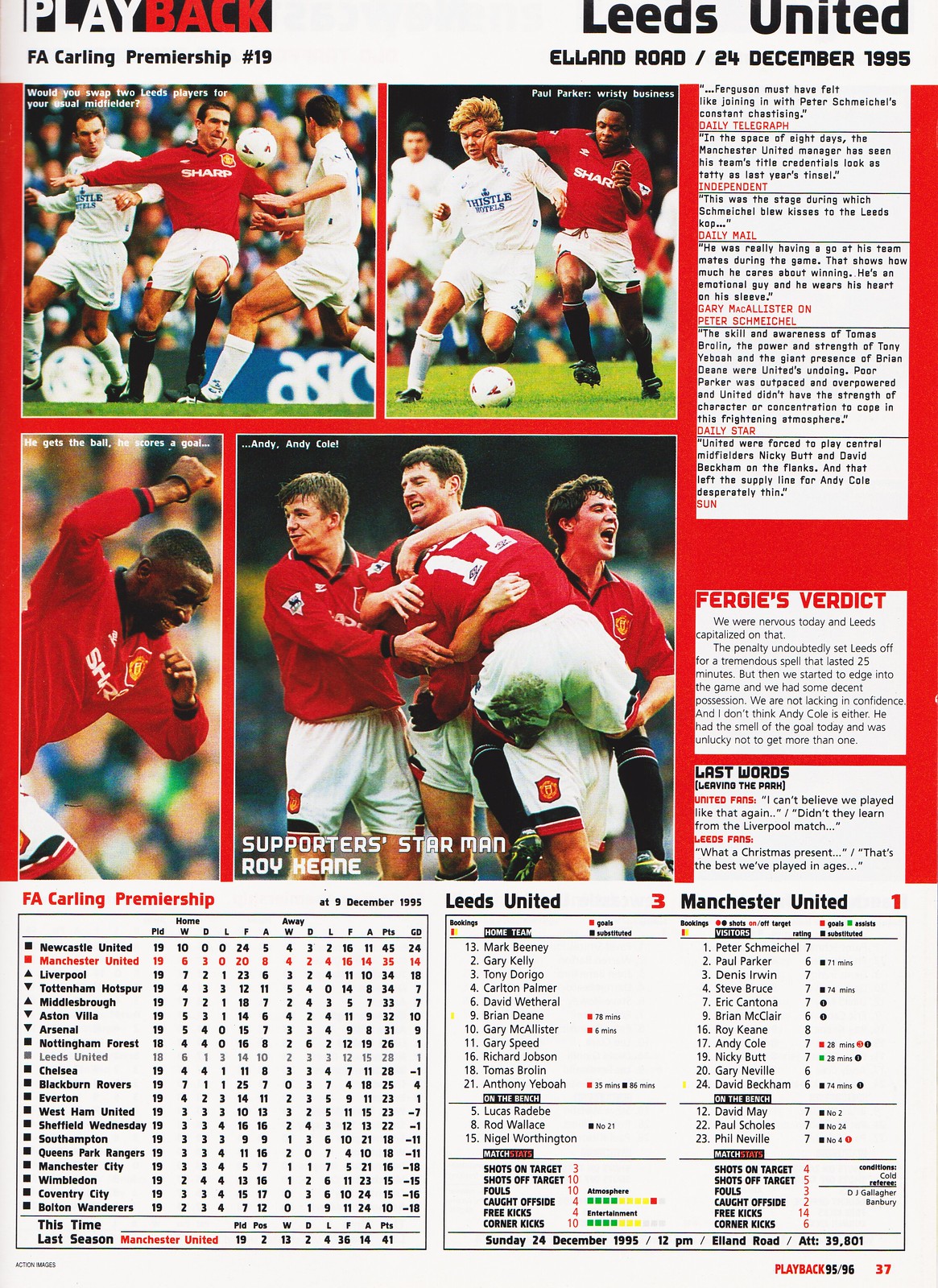The image resembles the front cover of a sports magazine, likely titled "Playback," and prominently features Leeds United. At the very top right, it reads "Leeds United" with the text "Elland Road, 24 December 1995" beneath it. The top left displays a black strip with the word "Play" in white text, followed by "Back" in red text just below. Below this, in black text, it reads "FA Carling Premiership, Number 19."

The layout includes four photographs depicting a match: in the first photograph, a player in a red shirt is handling the ball while confronted by an opposing team in white jerseys. Another image showcases a red and white player contesting and dribbling the ball. Both teams are wearing white shorts.

On the right-hand side, there are quotes from various publications, including the Daily Telegraph, Independent, Daily Mail, Daily Star, and The Sun. At the bottom, a chart displays the scores of the teams alongside the standings for the season, accompanied by statistics of different players.